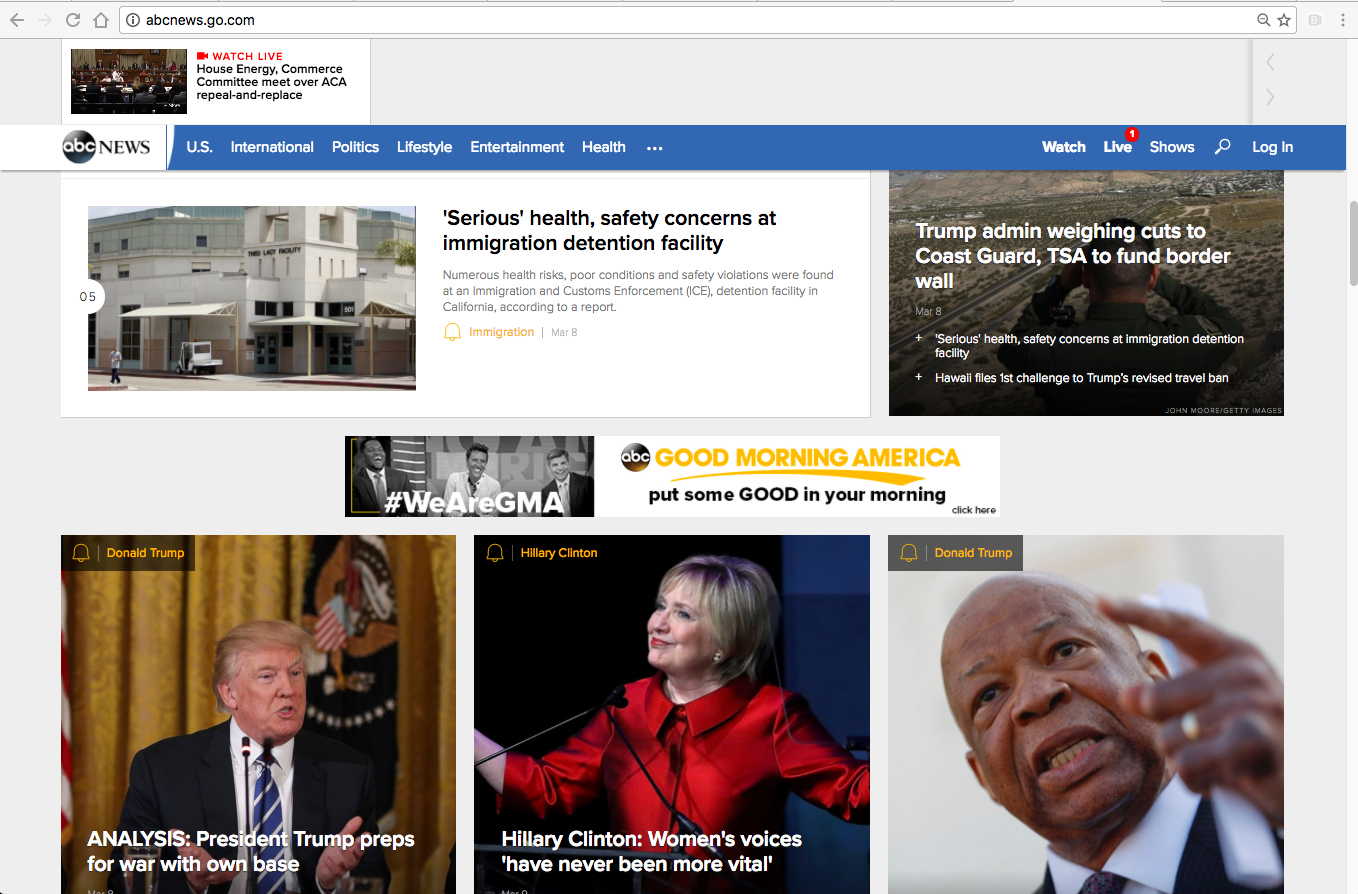This screenshot captures the homepage of the ABC News website, abcnews.go.com. The address bar at the top features a search and favorite icon aligned to the far right. Directly below, a bold red banner announces "WATCH LIVE: House Energy & Commerce Committee Meet Over ACA Repeal and Replace." The prominent ABC News logo is centrally positioned below this banner, with navigational links categorized under "US," "International," "Politics," "Lifestyle," "Entertainment," and "Health." Three white dots adjacent to these categories presumably offer additional options. To the right, there are icons for live streaming, search, and user login.

Below the navigation panel, the main news headline appears: "Health Concerns at Immigration Detention Facility." It details numerous high-risk conditions and safety violations identified at a U.S. Immigration and Customs Enforcement (ICE) detention facility in California, according to a report. This is followed by several other headlines: "Trump Administration Weighing Cuts to Coast Guard, TSA to Fund Border Wall," another study on "Health and Safety Concerns at Immigration Detention Facility," and "Hawaii First to Challenge Trump's Revised Travel Ban."

An advertisement for "Good Morning America" inviting viewers to "Put Some Good in Your Morning" is prominently displayed beneath these headlines. Following the ad are images accompanied by noteworthy headlines: a picture of President Donald Trump with the headline "Trump Preps for War With Own Base," an image of Hillary Clinton with the caption "Women’s Voices Have Never Been More Vital," and a final image featuring a black man in a suit pointing, identified as Donald Trump, but who is likely a congressman. However, his exact identity is unclear in this context.